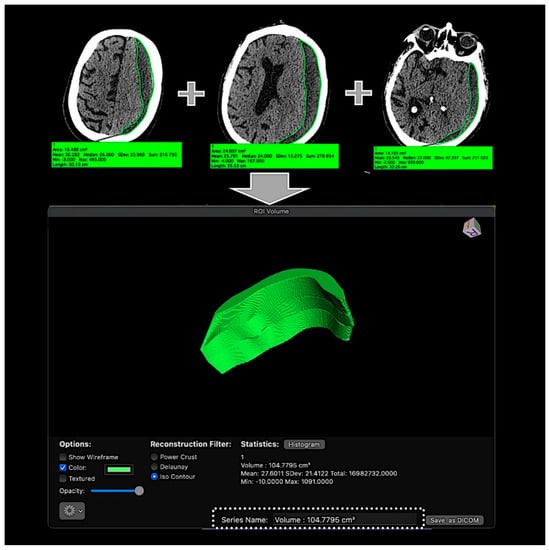The image displays a sophisticated medical program interface, possibly used by brain surgeons or neurologists, showcasing detailed scans of a human brain. Against a black background, the top section contains three cross-sectional views of a person's head, resembling MRI or CT scans, with distinguishable features like the outline of the brain and even the eyes. Directly beneath these scans, green text boxes—though too small to decipher—appear to provide supporting data. A prominent arrow points to a 3D model of an irregularly shaped, lime-green form, suggesting advanced imaging or reconstruction of brain activity or structure. At the bottom, legible text labels read "Options," "Reconstruction Filter," and "Statistics," indicating various analytical tools available within the software.